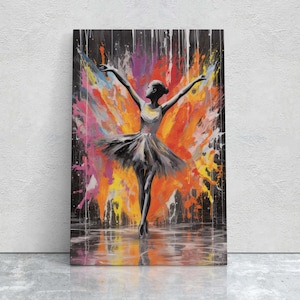The meticulously staged product photograph showcases a rectangular painting of a ballerina, presented against what appears to be a 3D-rendered white textured wall and reflective white marble floor. The ballerina, rendered primarily in black, grey, and white, is depicted standing gracefully on her tiptoes with her arms elegantly raised and head turned to her left. Behind her, an explosion of vibrant colors—orange, red, magenta, yellow, light blue, and white—contrasts vividly against a backdrop of black and white stripes. The reflective marble floor beneath the painting subtly mirrors the ballerina's figure and the color splashes, adding depth to the composition. The overall scene exudes a blend of abstract and realistic elements, highlighting the intricate details and vibrant colors of the artwork, making it a striking focal piece for any commercial setting.